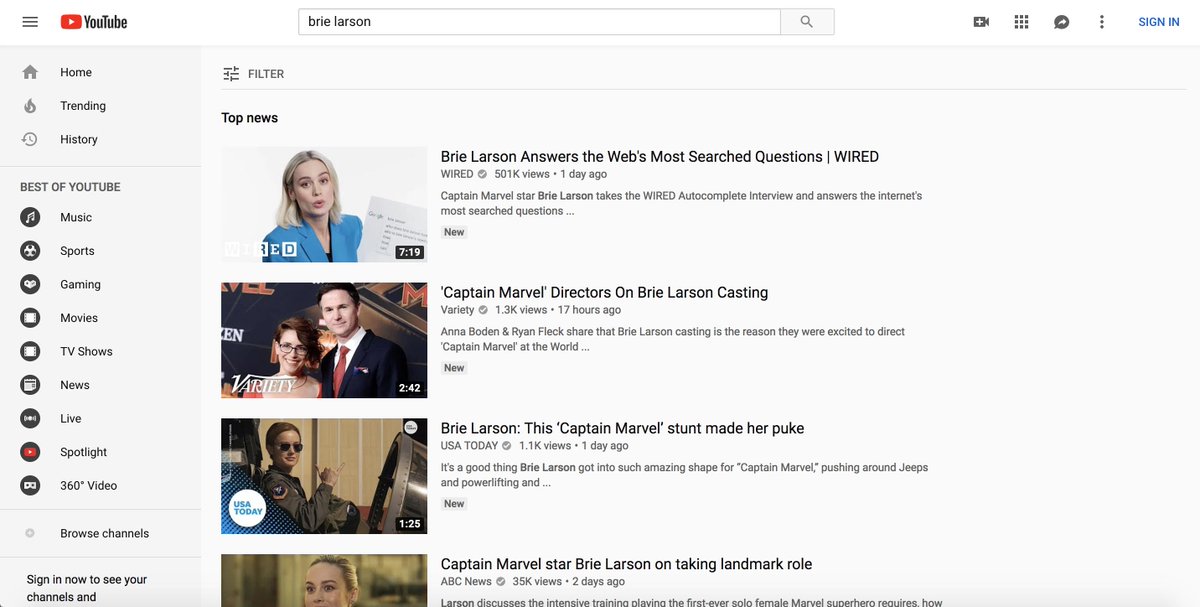This image is a snapshot of a slightly older version of the YouTube website as displayed on a desktop computer. In the upper left corner, you can see the signature hamburger menu consisting of three horizontal lines. Adjacent to this menu is the recognizable YouTube logo featuring the red play button. Central to the interface is a prominently placed search bar, with the name "Bry Larson" typed into it.

To the right of the search bar, additional user interface elements are visible, including a blue "Sign in" button, facilitating user login.

Dominating the center of the webpage is a list of video thumbnails. Each thumbnail includes a preview image on the left, with a duration timestamp in the bottom-right corner of the preview. For example, the first video displays a gray box with "7:19" in white text, indicating a length of 7 minutes and 19 seconds. Below each thumbnail, additional details are provided such as the video's creator (e.g., Wired), the number of views (e.g., 501k views), and the upload time (e.g., posted one day ago).

On the left side of the page, there's a vertical navigation menu featuring various categories users can select to explore different content areas. The categories listed are: Home, Trending, History, Best of YouTube, Music, Sports, Gaming, Movies, TV Shows, News, Live, Spotlight, 360° Video, and Browse Channels. There's also a prompt encouraging users to "Sign in now to see your channels," although the rest of the sentence is cut off.

Overall, this image captures the main elements of the YouTube interface, offering a clear view of its layout, search functionality, video listings, and navigation options.